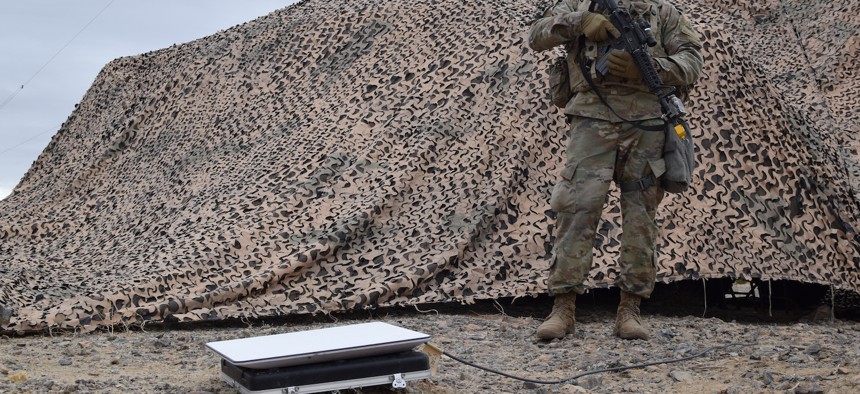In this daytime image, we see a clear sky on the left that transitions to clouds as we look further right. The scene appears to be set on a military base or similar outdoor setting, featuring rough gravel and a mix of brown and black rocks on the ground. Dominating the foreground is a large, camouflage-colored tent, displaying shades of beige, green, and brown. This tent stretches from left to right and seems to conceal or protect some type of equipment. In front of the tent, a soldier stands on the right-hand side, dressed in full camouflage fatigues, including brown boots and olive-colored, thick gloves. He’s holding a large machine gun pointed toward the ground with both hands, one finger resting near the trigger. The soldier also appears to be equipped with crossover bags on each side of his body. Near the tent, on the left-hand side of the soldier, there’s additional equipment—possibly a suitcase with a device resembling a solar generator, identifiable by a wire running into the tent. The soldier seems ready for combat, suggesting the area or equipment may need protection.